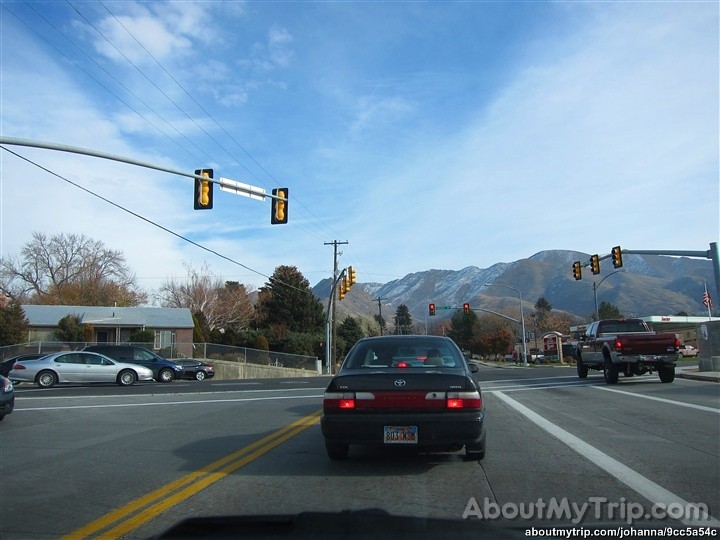The photograph, likely taken through a car windshield or dash cam, captures a bustling intersection with a unique criss-cross design where one road runs diagonally and the other meets it at a straight angle, creating an unusual visual perspective. Traffic lights are positioned at odd angles around this junction, and directly in front of the camera is a black Toyota with an Arizona license plate, indicating the setting is possibly Arizona. To the right is another car, also with an Arizona plate. Beyond the intersection, a house is visible on the left while a gas station is seen on the right. Mountains with snow-capped peaks, a vibrant blue sky streaked with white cirrus clouds, and a mix of healthy and barren trees create a picturesque backdrop. The photograph includes a watermark at the bottom right: "aboutmytrip.com," followed by a specific URL, "aboutmytrip.com/johanna/9cc5a54c," likely to track or view more of the trip's details.